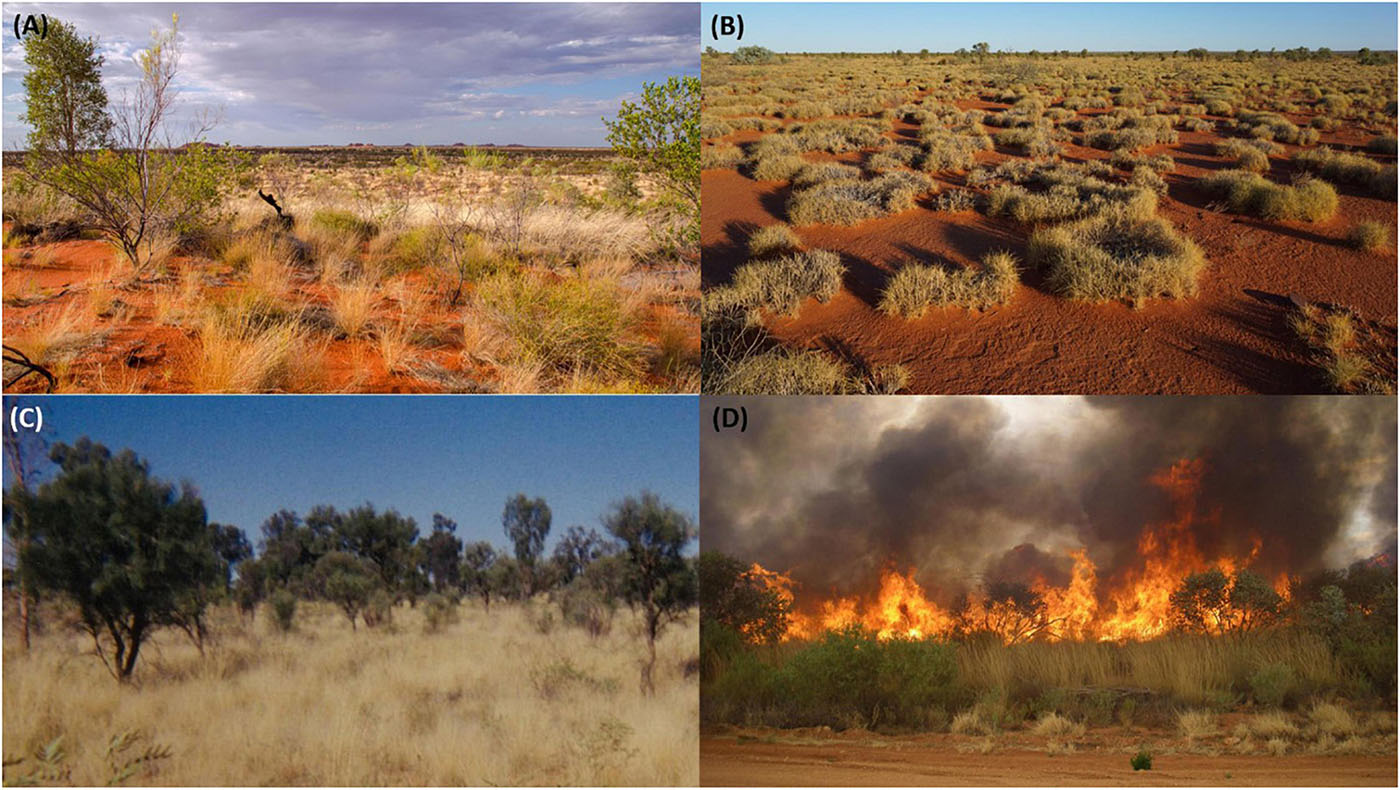This collage features four diverse landscapes, each meticulously labeled with black letters at the top right corner for clarity:

1. **Photo A** depicts a daytime desert scene marked by predominantly red soil. Sparse patches of grass intermittently cover the ground, while the sky is a clear, uninterrupted blue. Minimal trees dot the landscape, emphasizing the arid environment.

2. **Photo B** presents another daytime desert vista. This scene primarily consists of isolated bushes scattered across a parched terrain, under a bright, open sky. The vegetation is sparse, further highlighting the harsh desert conditions.

3. **Photo C** showcases a diverse daytime landscape featuring an uneven distribution of trees and brownish grass. The trees grow in a scattered pattern over the terrain, offering a glimpse into a semi-arid region.

4. **Photo D** captures a dynamic image of a fire during the day. Visible flames and rising smoke dominate the background, while the foreground reveals sparse grass and patches of bare red ground, mirroring the desert-like conditions seen in the other photos.